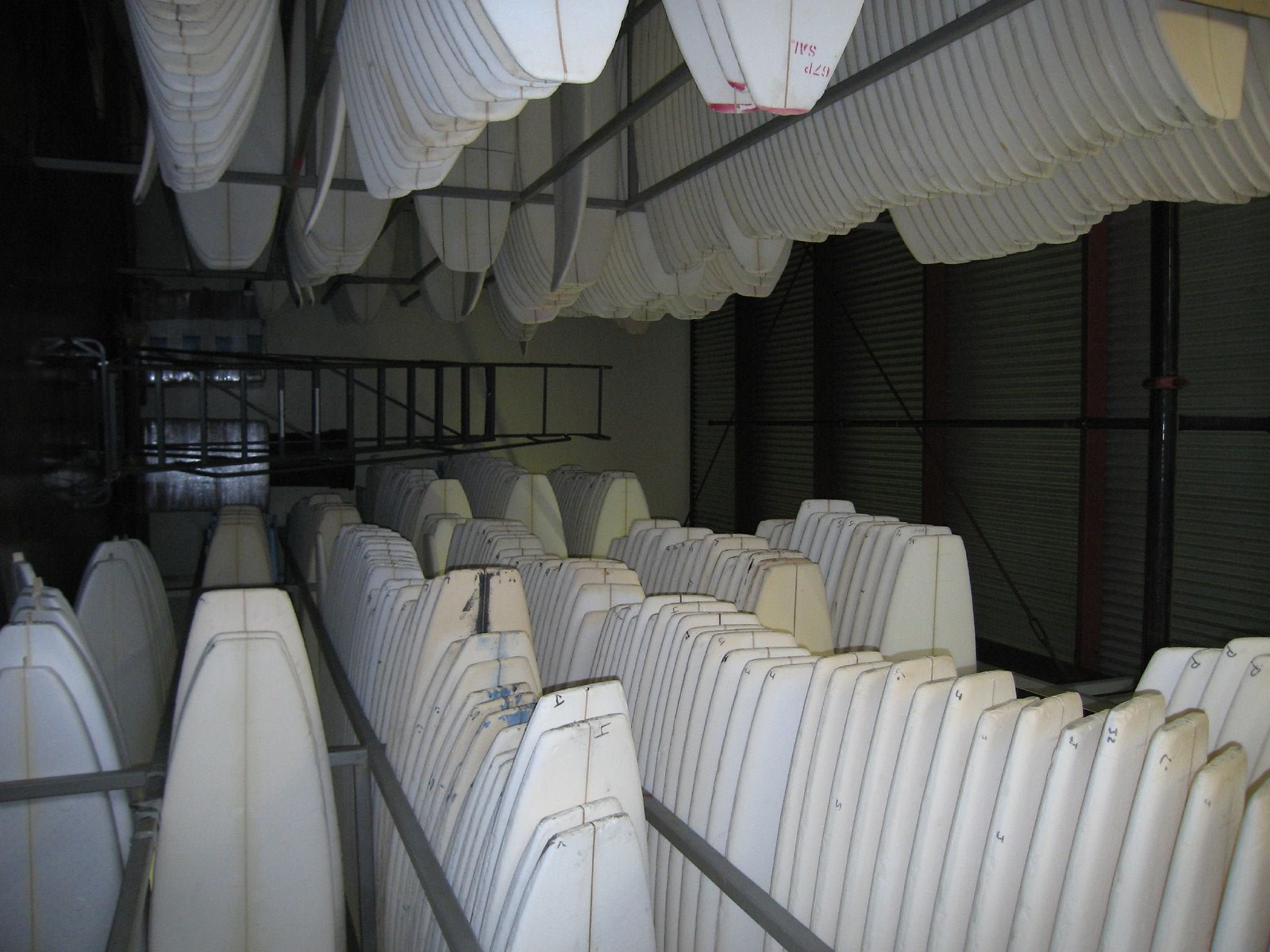This image captures the interior of a dimly lit surfboard manufacturing warehouse. The space is filled with an extensive array of white foam surfboards, all appearing to be unfinished blanks. These boards are predominantly lined up vertically in rows, each separated by dark gray or black metal bars and thin columns. The surfboards are densely packed, almost like dominoes, with several hundred visible both on the ground and suspended from racks overhead. The surfboards are arranged meticulously in numerous aisles that extend deep into the room, illustrating a highly organized system for storage. In the background, a horizontal ladder is affixed to the wall, which has corrugated steel panels and exposed beams. The room has windows with drawn blinds and a mix of dull silver and possibly yellow metal racks, contributing to an industrial aesthetic. Despite the warehouse's darkness, the stark white surfboards stand out, creating a striking monochromatic scene devoid of any text or notable coloration.